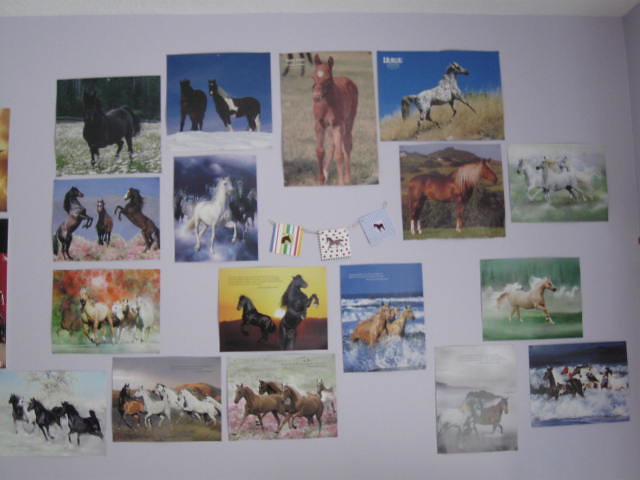Displayed on a bluish-gray wall that might be part of a young girl's bedroom, there's a captivating collection of approximately 15-20 horse-themed photos. These images depict horses in a variety of scenes and positions—some are standing still, while others are galloping majestically, trotting up hills, or splashing through water. The horses in these photos are of diverse breeds and colors, including white, black, brown, and speckled coats. Noteworthy scenes include three horses rearing up against each other, two horses running through the ocean waves, and a drawing of a white horse. At the center of this arrangement, there's a decorative string adorned with three small square banners, each featuring horse graphics. The wall also features horses in different environments: grassy meadows, snowy fields, and sunny landscapes. This array of imagery, some possibly movie scenes while others appear to be nature photographs, underscores the owner's profound love for horses, making it a vibrant equestrian tribute.